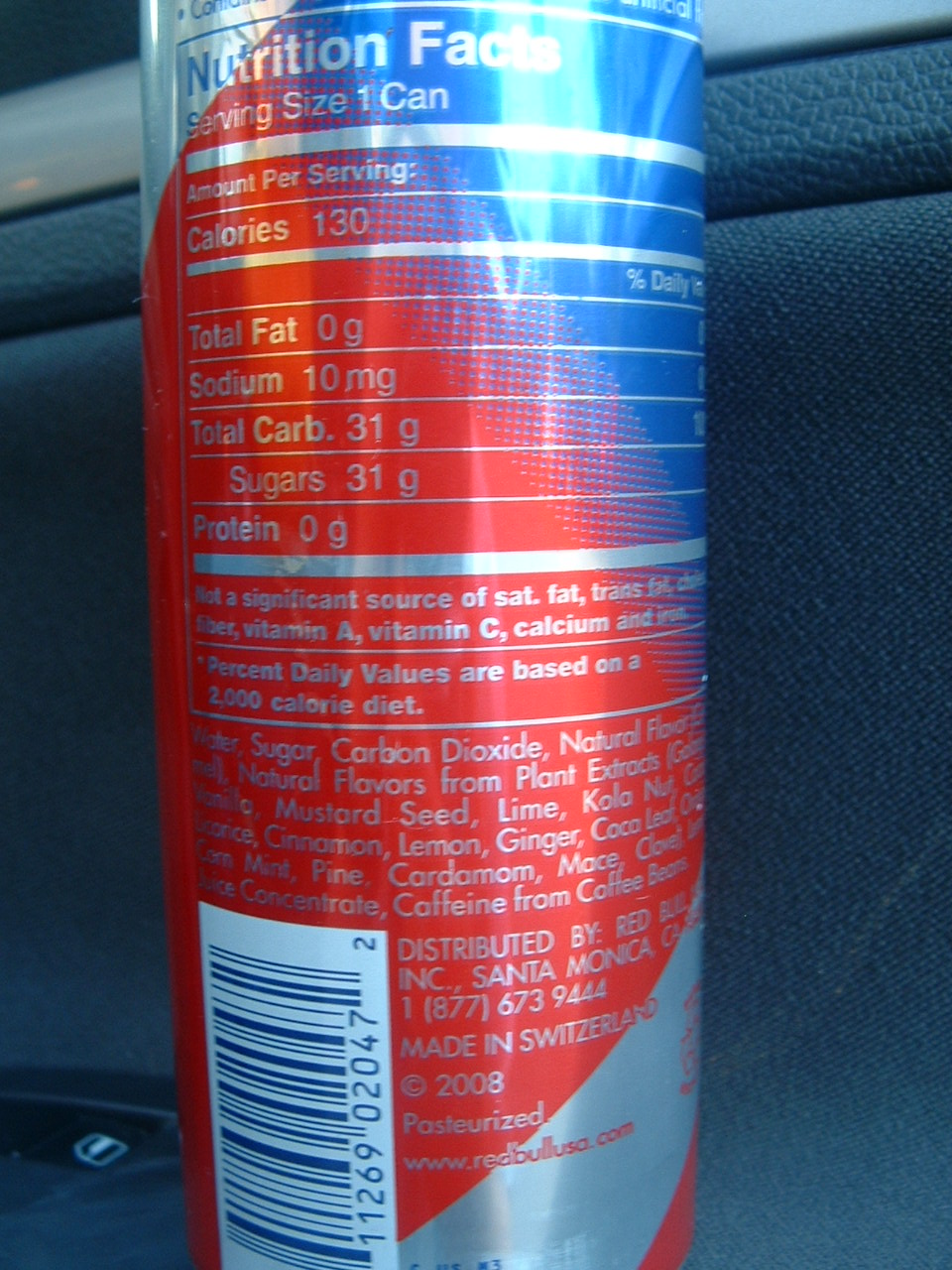This image showcases the back of a beverage can, prominently featuring nutritional information, serving size, and calorie content, suggesting it is a drink. The can's design is predominantly red, with a silver stripe ascending from the left-hand side, resembling a ribbon that wraps around the can and emerges at the top left. The design also incorporates sections of blue, alongside an intricate pattern of red and blue dots. A large barcode is visible on the bottom left-hand side, but the specific type of drink remains indeterminate due to the partially obscured text and graphics.